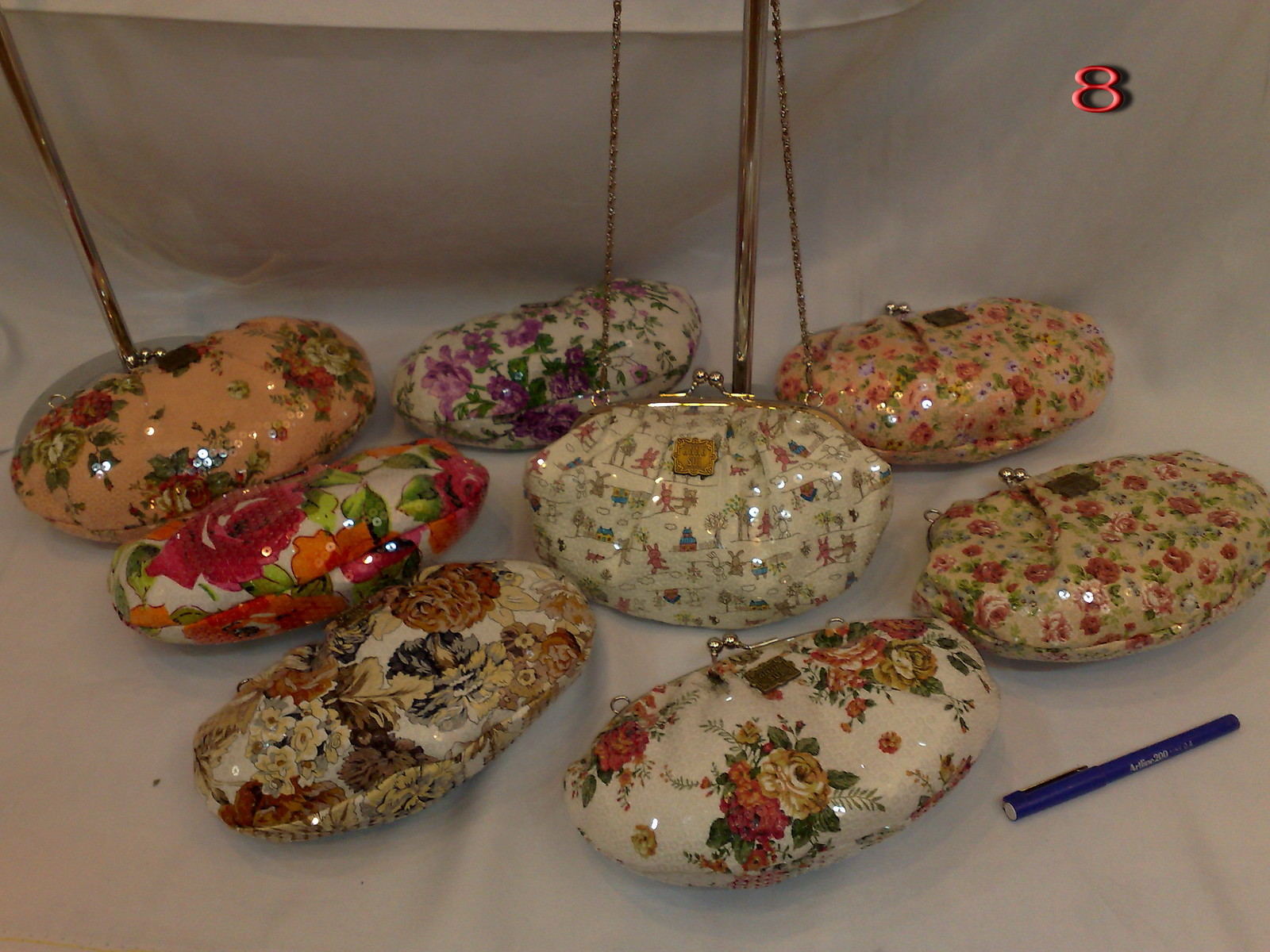This color photograph features a close-up of eight intricately patterned coin purses laid out on a white cloth background. Each purse is adorned with a floral design, reminiscent of vintage styles typically associated with Grandma Gertrude's aesthetic. The purses are primarily composed of a harder material, possibly resembling clamshells, and embellished with sequins. Each one is equipped with a twist-lock clasp featuring gold balls and long gold chains. The arrangement starts from the top left corner and proceeds rightward, then down the rows.

In the top right corner of the photograph is a red number 8, casting a shadow behind it. The purses vary in their color schemes and floral decorations. One purse is a peachy beige with red roses and green leaves, another is cream-colored with pink roses, and a third features a pattern of purple flowers on a white base. Further variations include a cream background with small frolicking rabbits amid houses and trees, and another with mauve-colored roses and sage green leaves on a yellowy cream base. There are autumn-themed designs with burgundy, navy, and cream hues resembling pine cones. Prominently, front and center of the arrangement is a cream background purse with gold and mauve red roses. 

Additionally, a blue pen with a white top lies in the front right corner of the setup, adding a casual, everyday element to this otherwise ornate grouping.